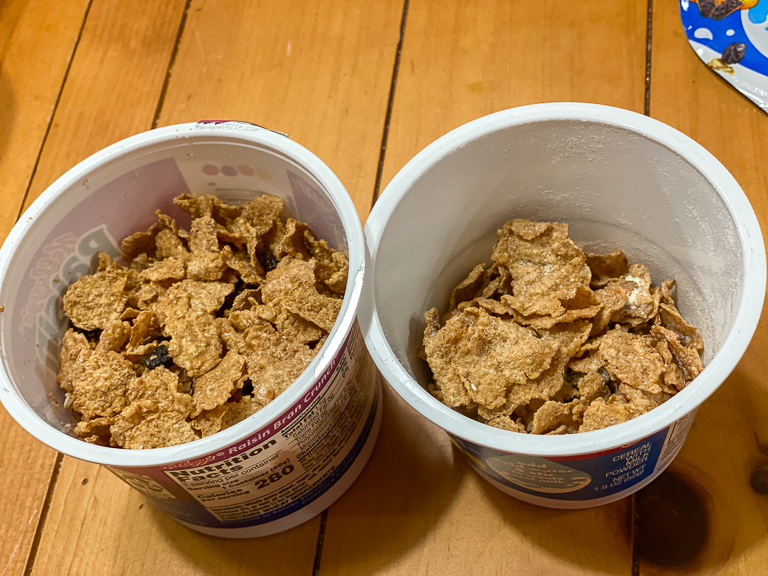The image features a top-down view of two plastic containers on a wooden table with brown planks. Both containers are filled with brown Raisin Bran cereal, identifiable by the visible raisins mixed in with the bran flakes. The container on the left prominently displays the nutrition facts, including a calorie count of 280, and is about two-thirds full. The container on the right, roughly one-third full, has partial text indicating "cereal with milk," though the full label is obscured. One container is from Kellogg's Raisin Bran Crunch, aligning with the cereal's appearance. The setting and packaging details highlight the wastefulness of single-use plastics.